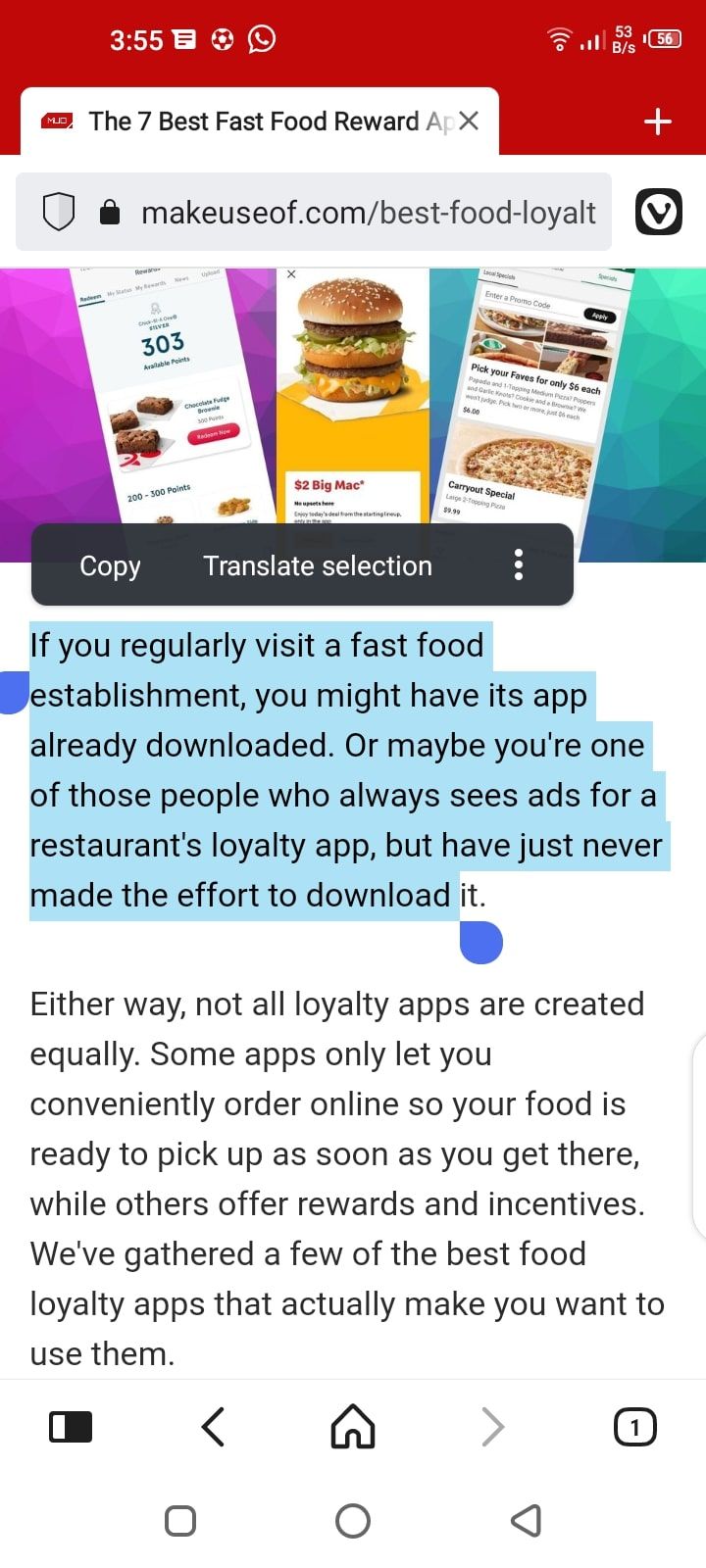A vibrant and busy smartphone screenshot filled with a multitude of apps and notifications. At the center, a weathered hand holds a soccer ball, bordered by a semi-transparent bubble. The background is predominantly red, accentuated with various icons such as a Wi-Fi symbol displaying three bars, and a battery icon showing 56% charge. Additionally, there is a progress bar marked 'red' and black text stating "The 7 Best Fast Food Rewards."

Prominent in the interface is the website address makeuso.com displayed upside down, with a shield and lock icon nearby, indicating security. A rectangular section toward the left is shaded in purple and is labeled with '303,' adding to the informational overload. Below this, a stacked Big Mac is showcased against a white background that transitions to yellow at the bottom. A slice of pizza is also visible alongside more text in blue and gray shades.

The screen features continuous and engaging commentary about fast food loyalty apps, highlighting the benefits and functionalities of the apps. "If you regularly visit fast food job sites, you might already have this app downloaded," the text reads, drawing attention to the usefulness of such applications. Further text, emphasized in the background, elaborates on the unique features and rewards these apps offer.

The left side of the screen is adorned with a bar, while the right side reveals a glimpse of a building. The top section of this crowded screenshot includes a square icon, adding to the array of visual elements. Overall, the image encapsulates the digital clutter commonly seen on active smartphone screens, emphasizing the theme of fast food loyalty applications and their advantages.